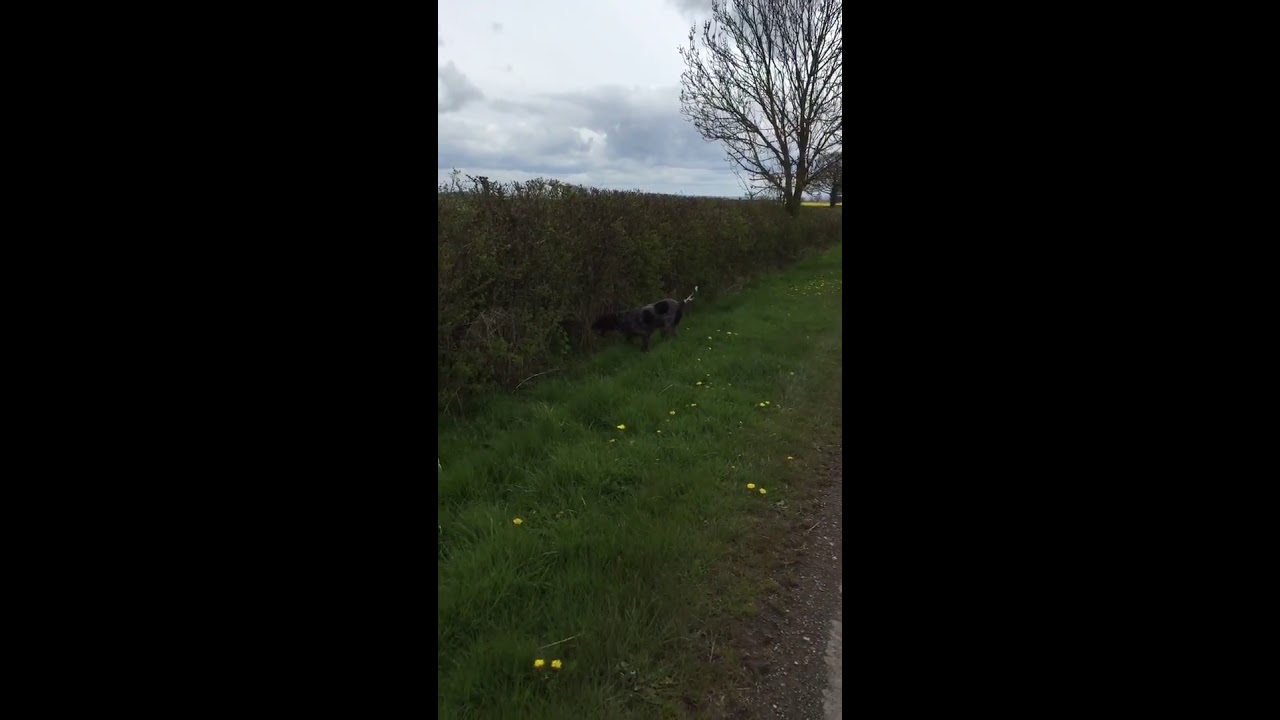In this detailed outdoor photograph, a gray and black hound-like dog traverses an overgrown grassy field during daylight. The field, lush but unkempt with ankle-high greenery, features scattered yellow buttercups. A tall hedge of bushes, trimmed to resemble a wall and about six feet tall, runs along the left side, while a partly bare-branched tree stands prominently in the foreground to the right. The horizon reveals a backdrop of sparse trees, hinting at the fall season. Mud and sand can be seen near the grassy area, indicating a nearby road. Overhead, the sky is a mix of blue and white, filled with puffy clouds, enhancing the serene yet wild nature of this countryside scene.